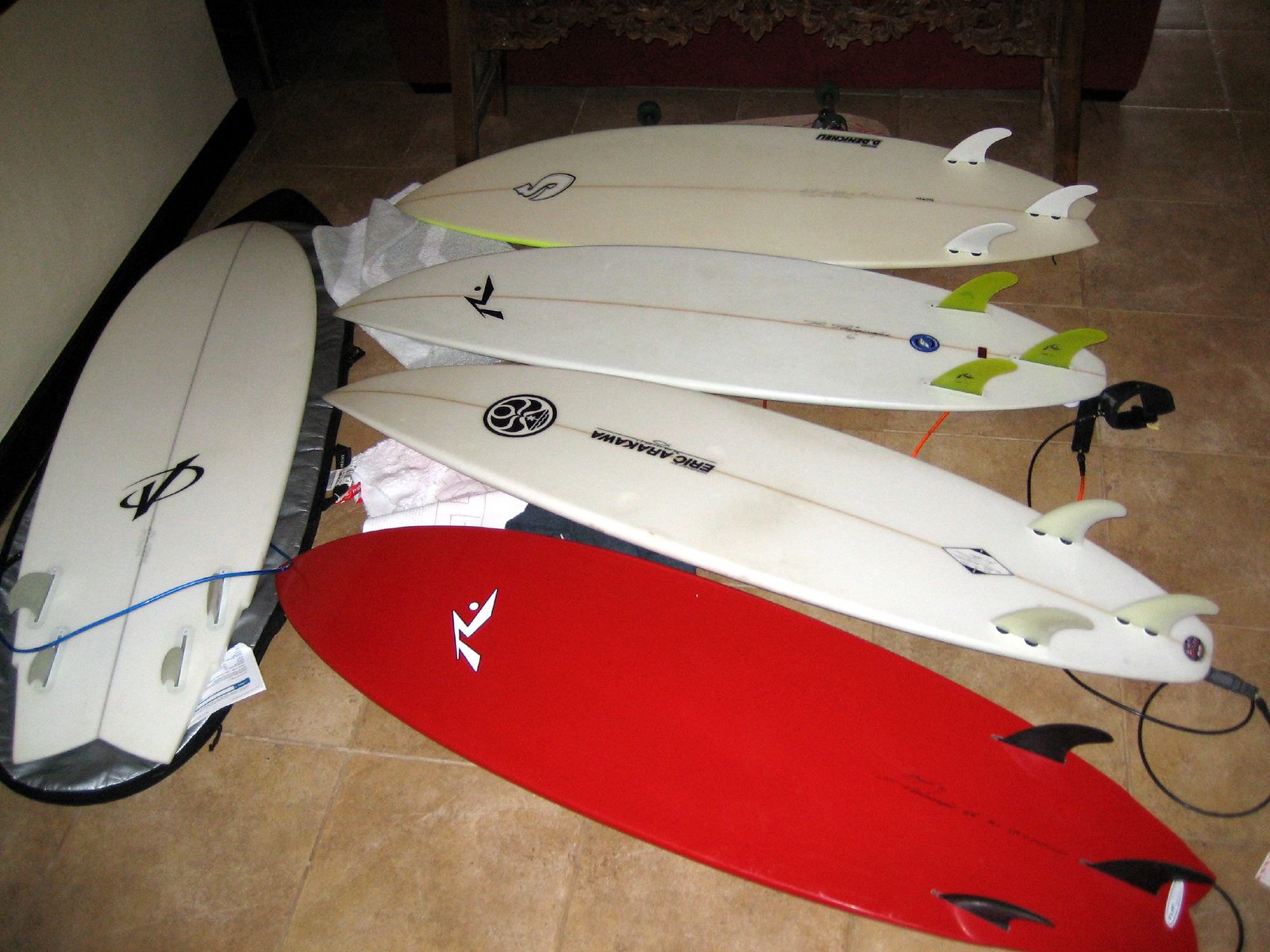The image shows five surfboards arranged on a tiled floor in what appears to be an indoor room, possibly a mudroom or garage. Four of the surfboards are white, and one is red. The red surfboard, closest to the viewer, has black fins, while among the white surfboards, one has green fins and the others have white fins. Four of the surfboards are laid out horizontally in a straight line, with an additional one positioned vertically to the left. Notable branding includes "Eric Arakawa" on at least one surfboard. Additional items in the scene include some cabling, a case under one of the surfboards, and some towels underneath the further surfboards, suggesting a casual, storage-like setting.